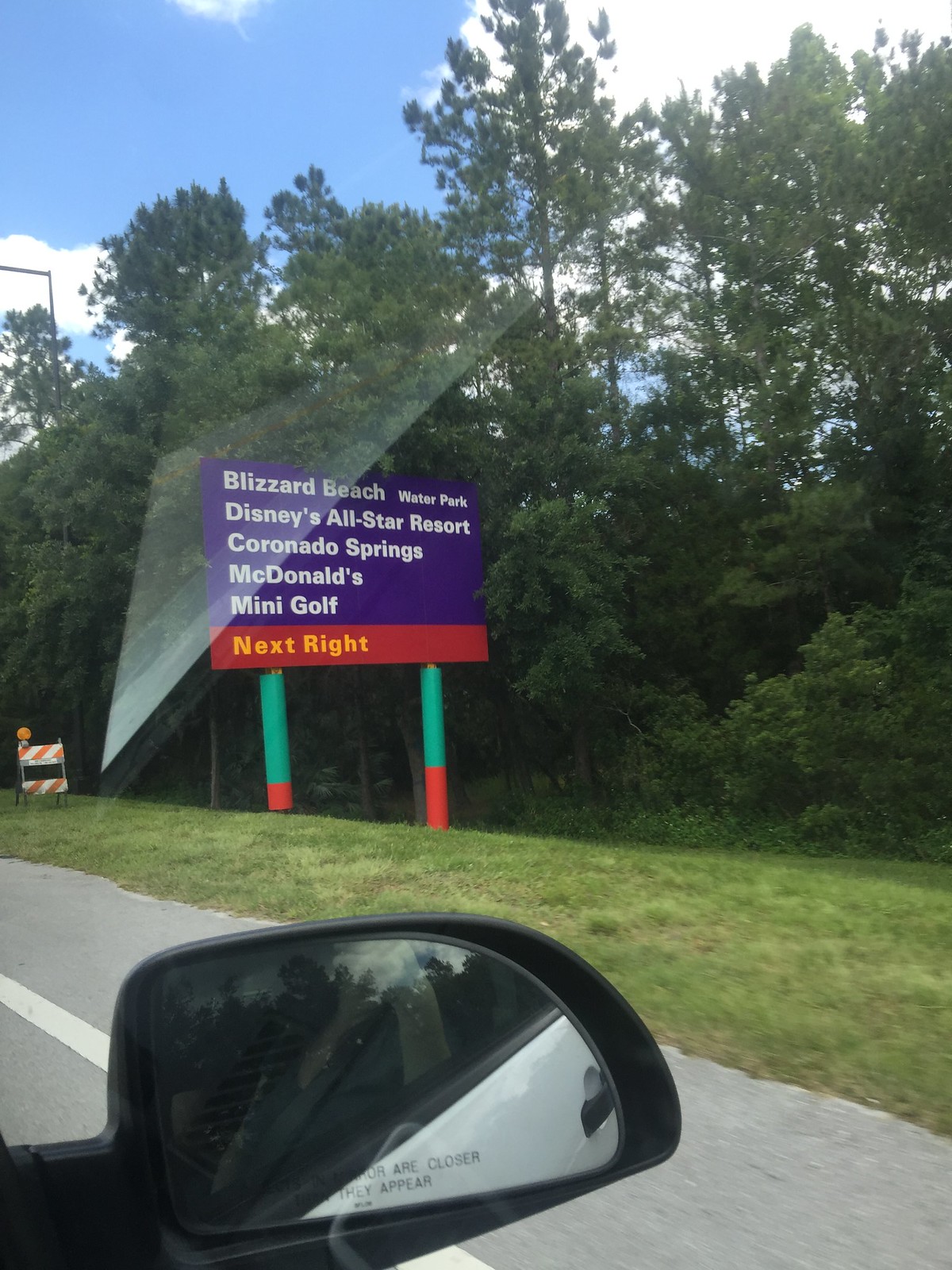The photograph, taken from inside a car on the right side and focusing out the front passenger window, highlights a detailed road scene. Prominently framed at the bottom left corner is the car’s right side view mirror, reflecting part of the car's light-colored body and a bit of the passenger window. Surrounding the mirror, the gray pavement extends to a freshly mowed grassy patch situated off the road's edge.

The main focus of the image is a multi-colored road sign near the grassy area. The sign, supported by green and red legs, features a blue background with white lettering that reads: "Blizzard Beach Water Park, Disney's All-Star Resort, Coronado Springs, McDonald's, Mini Golf." Beneath this, a red banner with yellow lettering states, "Next Right." 

Behind this sign, a tall tree line stretches across the frame, contrasting against the clear blue sky and scattered white clouds visible at the top left corner. Additionally, a small wooden trifold hazard sign with orange and white stripes, topped with a round orange flashing light, sits on the grass to the left of the main sign, completing the detailed and vibrant scene of the highway surroundings.